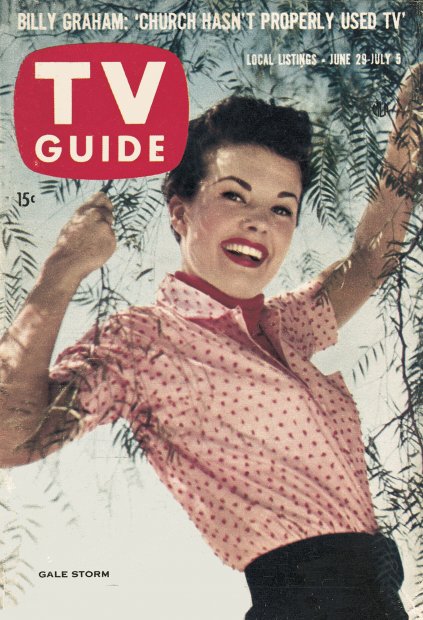The image is the front cover of a vintage TV Guide magazine, prominently featuring a poised and smiling woman named Gale Storm at its center. She has fair skin, bright red lipstick accentuating her smile, and her dark, shorter hair is neatly styled. Gale is dressed in a white blouse adorned with a pink polka dot pattern and pairs it with a black skirt or high-waisted pants. Her eyebrows are well-groomed, adding to her polished appearance. In the background, there is a tree with visible branches and leaves, indicating she might be casually swinging from it.

The top left corner of the cover displays the iconic TV Guide logo in white text against a red backdrop, resembling a television screen. Above Gale’s name, which appears in small black text on the bottom left, there is a white text caption that reads, "Billy Graham: Church hasn't properly used TV." Below this caption, the issue dates are listed as "Local listings, June 29th through July 5th." The overall style and elements suggest a classic 1950s aesthetic, with Gale Storm being the main focus of this engaging magazine cover.